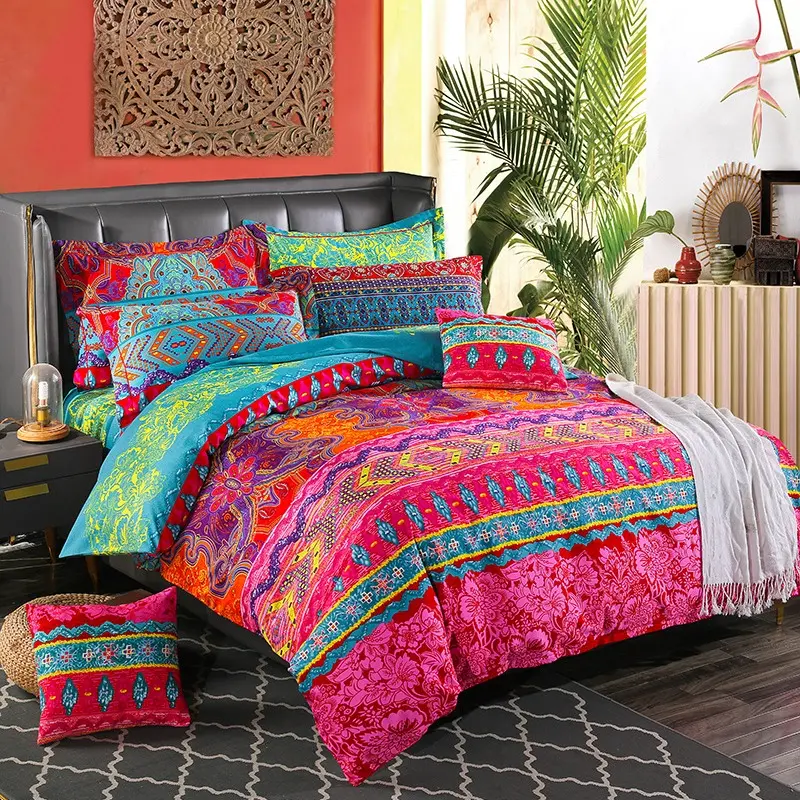This detailed photograph, likely taken in a showroom for a catalog, depicts a meticulously staged designer bedroom designed to showcase various pieces of furniture and textiles. Central to the scene is a full-sized bed adorned with a vibrant, multi-colored comforter featuring an intricate pattern of large pink floral stripes, small mosaic blue stripes, and pink stripes with blue diamonds. The bed is framed by a plush black leather headboard and flanked by four matching pillow shams with two additional pink throw pillows—one is positioned on the bed, while the other lies on the dark hardwood floor beside it.

A light gray blanket or scarf with fringe detailing is draped casually over the right corner of the bed. The bed rests on a dark hardwood floor partially covered by a gray carpet. On the left side of the bed, there are a couple of throw pillows on the ground and a dome-shaped candle holder containing a lit candle. 

A large indoor palm plant stands tall to the right of the bed, nearly reaching the ceiling and adding a touch of greenery to the room. Next to the plant, a small chest of drawers houses a couple of ceramic vases and a jewelry box on top, emphasizing the room's designer aesthetics. Above the bed, a wooden wall hanging with an Aztec-inspired design of interconnected circles is mounted on an orange background, providing a striking focal point. In the background, a wooden side table complements the room's decor, featuring additional vases and a wooden mirror. 

This 8-inch by 8-inch photograph captures the elegance and detail of the room, highlighting its well-coordinated color palette and thoughtfully selected decor, with no text or other features present in the image.